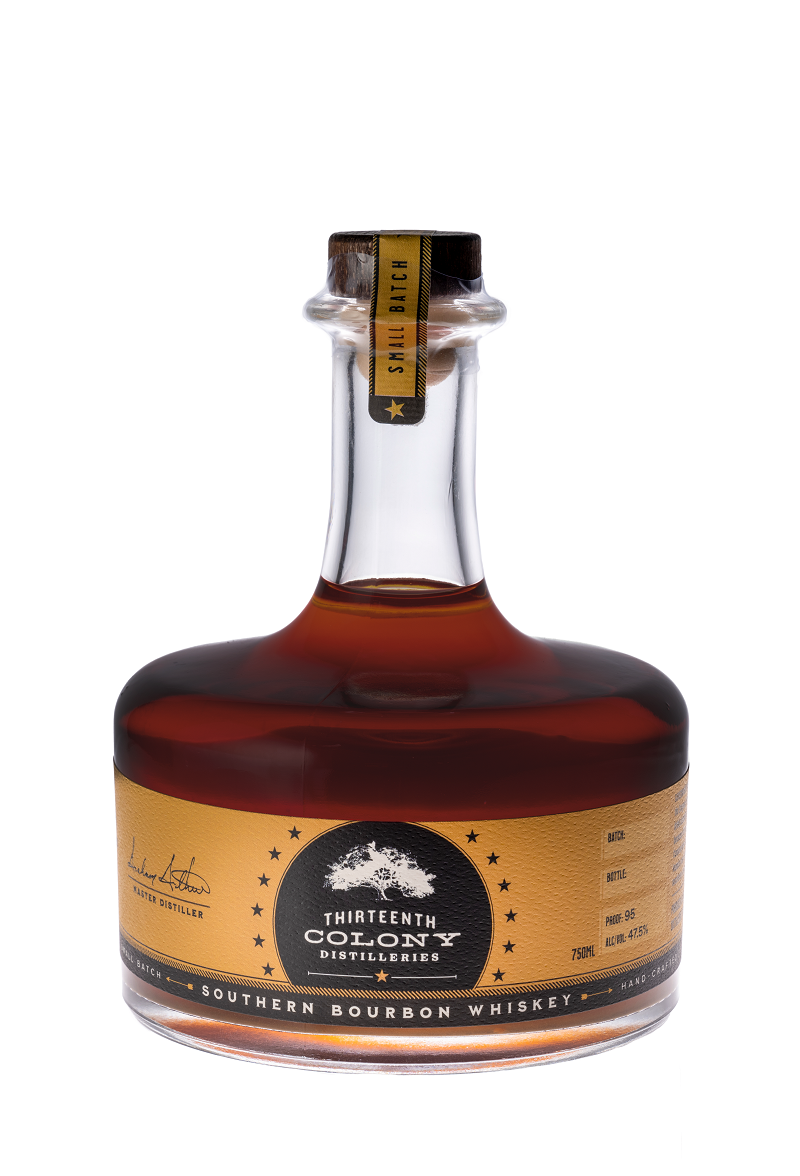This image showcases a distinct bottle of Southern Bourbon Whiskey from 13th Colony Distillers, set against a plain white background. The clear glass bottle, filled with a rich amber liquid, features a wide and stout shape that narrows at the neck. Its upper neck is topped with a black cap sealed with black and gold, which is unopened. The neck and cap are adorned with a label that reads "small batch," accompanied by a yellow star. The main label on the bottle’s body is tan with a black circle logo featuring the 13th Colony Distillers name and a white tree icon. Below this, in clear text, it states "Southern Bourbon Whiskey." The bottle is notable for its uniqueness, such as the design details and the prominent placement of the brand's imagery and text.